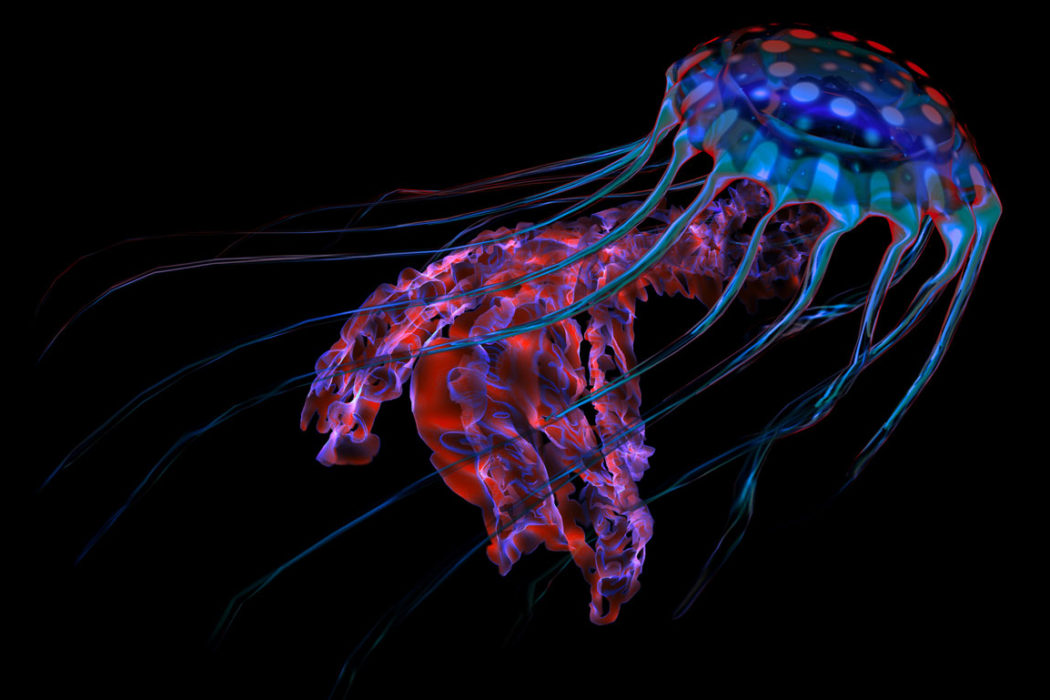The image depicts an AI-generated art piece on a black background, featuring a glowing, vibrant sea creature that combines attributes of a jellyfish and an octopus. Dominating the upper right corner is a circular, dark blue shape adorned with lighter blue spots at the front and red spots towards the back. This shape seamlessly transitions into tentacle-like appendages with a melty effect. These tendrils, ranging from thicker red and blue ones at the center to thinner greenish-blue strands extending leftward, create an octopus-like appearance. The central part of the creature features crinkly ribbons that add texture, glowing with vivid shades of purple, pink, and red. The overall luminescence of the creature's bright, almost neon colors—including dark blue, light blue, red, and silvery blue—stands out dramatically against the dark backdrop, capturing attention with its mesmerizing, otherworldly beauty. The sea creature's many tentacles seem to envelop a mysterious, vaguely humanoid red shape, adding an element of intrigue to this captivating composition.